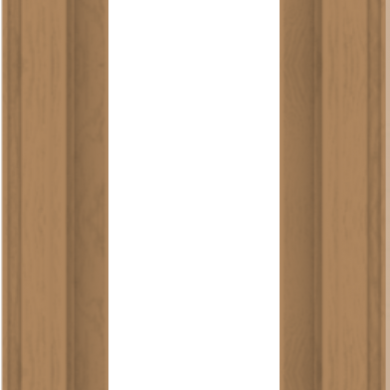The image displays a somewhat indistinct design composed of three vertical sections. Flanking both the left and right sides are pieces of tan-colored, wood-grain paneling with a matte finish. Both pieces have a varied grain pattern with stripes of different shades, suggesting imitation hardwood flooring. The left panel transitions from light tan at the top to darker hues towards the bottom, and the right panel inversely starts darker on top then lightens downwards. The center section of the image is a plain, wide white strip, devoid of any texture or features, starkly dividing the two wood-grain panels. The overall arrangement gives the impression of three vertical columns laid side by side, with two sections mimicking stained wood that aren't particularly glossy, and a blank white space in between.